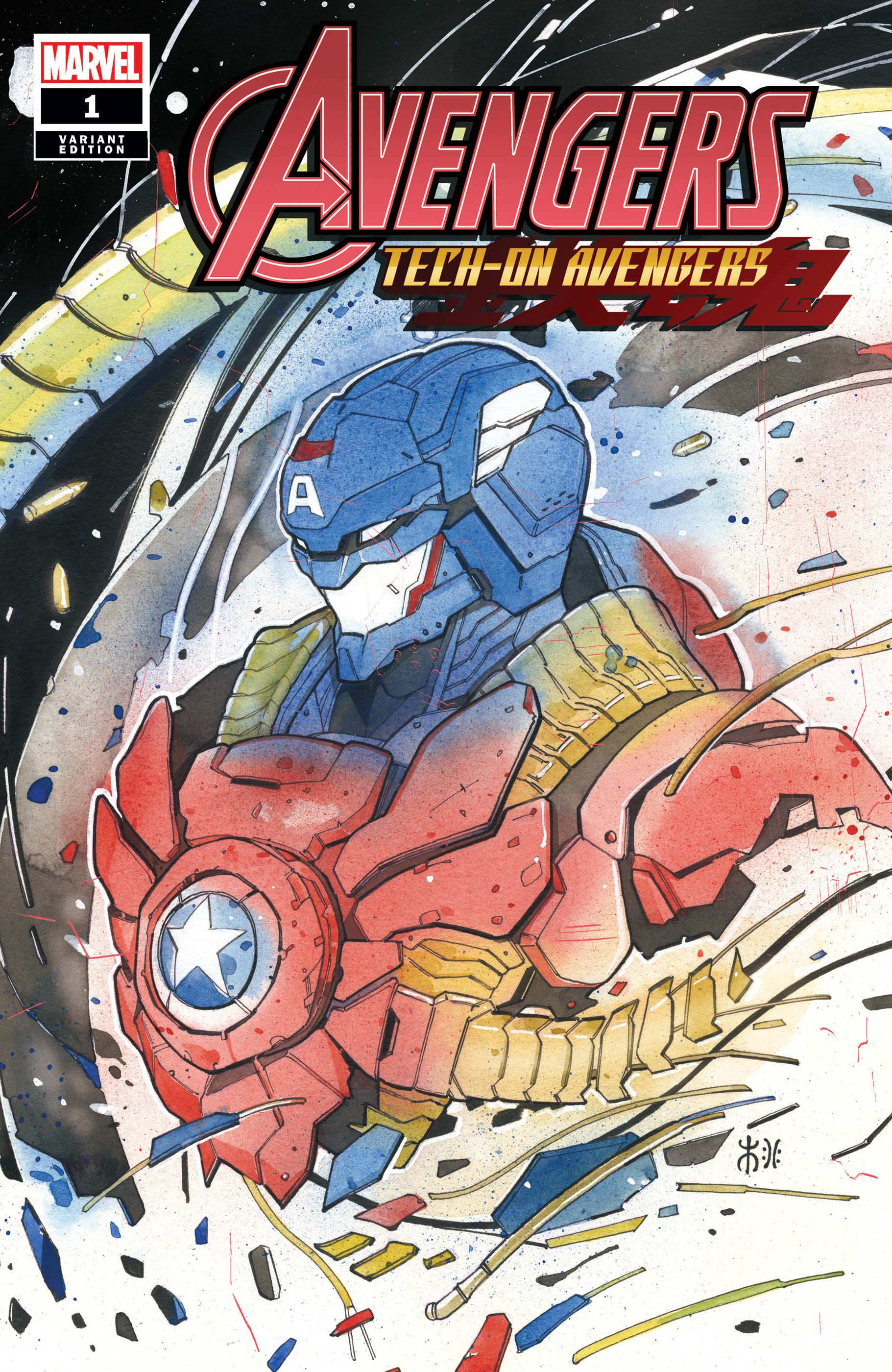This is a detailed poster for the first edition Marvel comic book, "Avengers: Tech-On Avengers." At the top, the Avengers logo is prominently displayed in red with the subtitle "Tech-On Avengers" in a distinctive orange-yellow. The top left corner notes "Marvel" and "One Variant Edition" in white text on a black and orange background.

Central to the poster is a tech-enhanced rendition of Captain America, featuring a blue helmet with a white "A" prominently on the forehead. His eyes appear to be glaring intensely, and the mouth area is white with a red outline on the jawline. His uniform is a striking mix of colors: deep reds, vibrant yellows, and blues. Yellow straps extend over his shoulders and connect to a central chest plate, which is red with a prominent blue circle and a white star in the center. Surrounding Captain America, the background is a stark black with scattered white and multicolored elements, giving a dynamic contrast to the detailed, deteriorating tech elements swirling around him, which appear like debris breaking away from his form. The overall impression blends the traditional superhero aesthetic with high-tech, almost mechanical details, enhancing the visual impact of the cover.